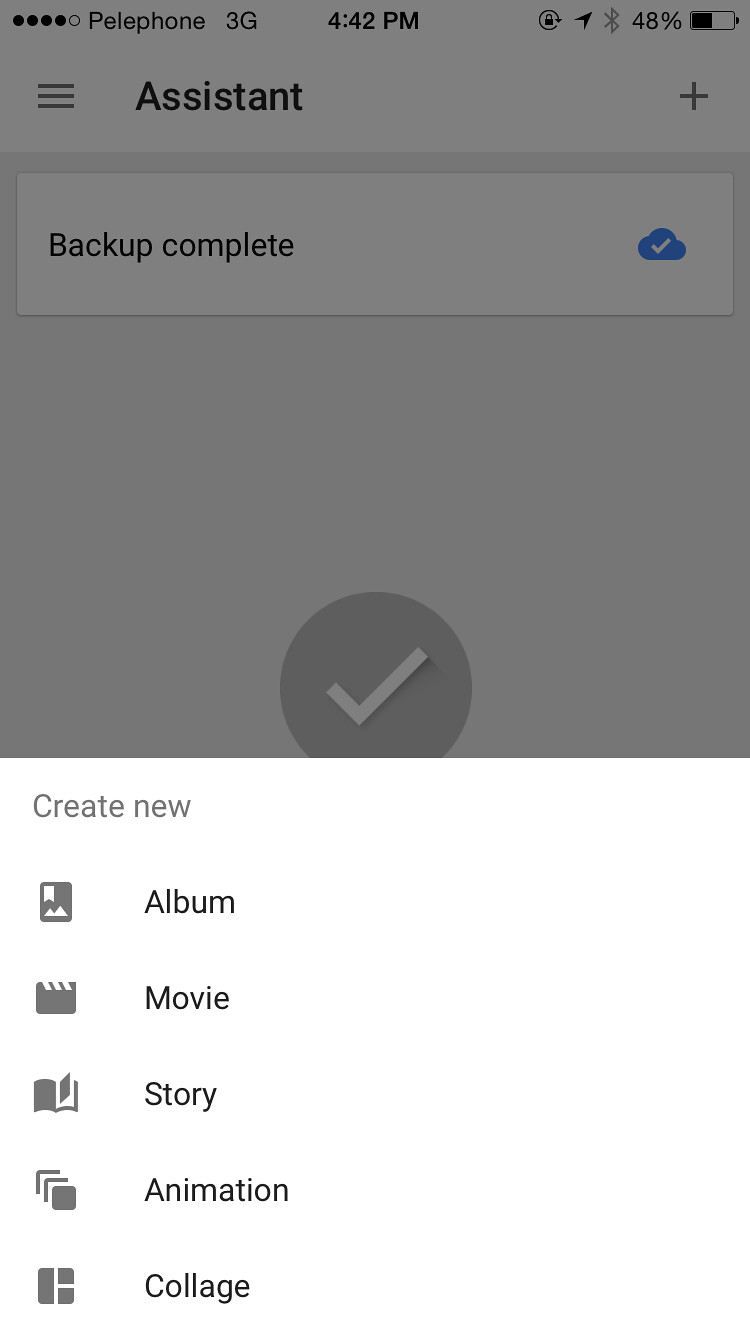This image is a screenshot depicting an interface of what appears to be Google Cloud or a similar online backup service. The top portion of the screen is shaded in dark grey, while the lower section is primarily white with text displayed in a very dark grey or black font.

In the bottom section of the image, the options "Create New Album," "Movie," "Story," "Animation," and "Collage" are listed, each accompanied by a respective icon. The "Album" icon is a small rectangle featuring mountains, the "Movie" icon resembles a clapperboard, the "Story" icon looks like a book with open pages, the "Animation" icon shows a series of squares placed diagonally atop one another, and the "Collage" icon is depicted by an arrangement of a long rectangle and two smaller squares.

Above this section, a slightly greyed-out area displays the word "Assistant" on a white bar that spans the entire width of the screen. This white bar contains three small horizontal lines in the top left corner and a plus sign in the top right corner.

Further up, another white bar reads "Backup Complete" alongside a blue cloud icon with a tick mark, also stretching across the full width of the screen but consuming about 10% of the vertical space. Right in the center of this greyed-out top section, there is a prominent grey circle with a white tick mark inside.